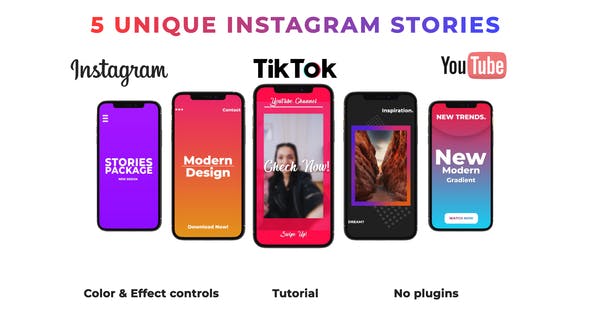This image, sourced from Instagram, features a compilation of five unique Instagram stories. Positioned on the left, the word "Instagram" is elegantly written in black cursive print. Centrally located is the word "TikTok," also in bold black lettering. To the right, "YouTube" is prominently displayed with the 'You' in capital letters and 'Tube' encased in a red TV screen graphic.

At the bottom of the image, the words "Color and Effect Controls" appear on the left, a central "Tutorial" label, and "No Plugins" written on the right. Between these phrases, five smartphones are arranged in a tiered display—highlighting various Instagram story templates.

The largest smartphone, positioned beneath "TikTok," showcases a medium-sized template labeled "Check Now." Flanking this phone are two medium-sized smartphones; the one on the left displays "Modern Design," while the one on the right presents an unspecified image.

Lastly, the smallest phones are located beneath the "Instagram" and "YouTube" labels, displaying "Stories Package" on the left and "New Trends, New Modern Confident" on the right. This detailed arrangement emphasizes various design options available for creating engaging Instagram stories.